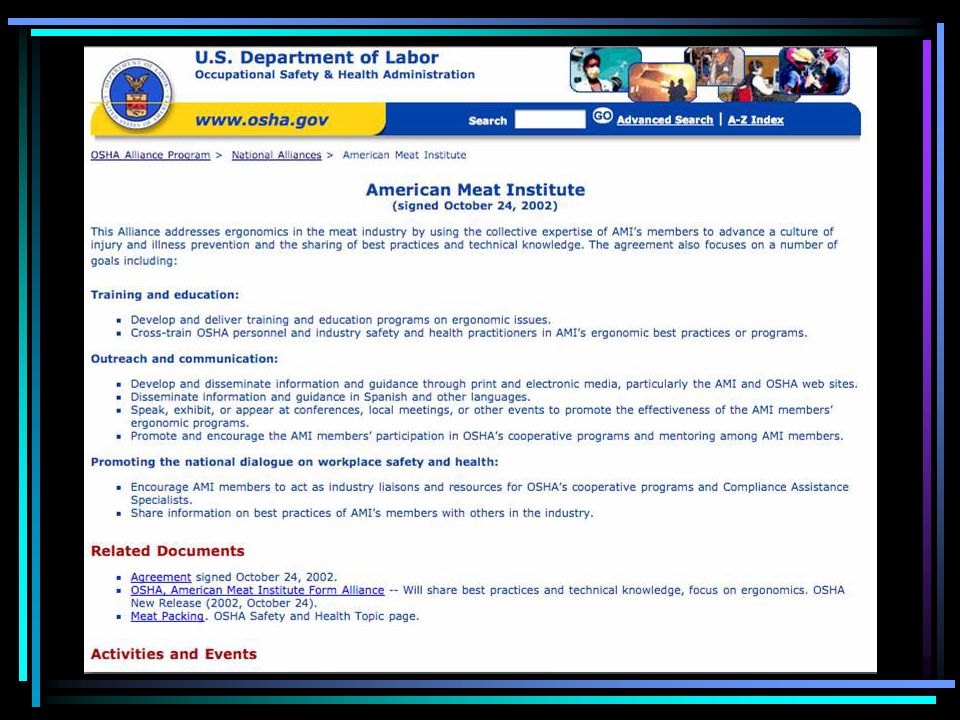The screenshot captures a vivid and detailed view of the U.S. Department of Labor's Occupational Safety and Health Administration (OSHA) website. The interface is unexpectedly vibrant, adorned with a colorful banner featuring hues of purple, teal, and light blue, which add an engaging touch to the page. 

At the top center is the distinguished seal of the U.S. Department of Labor, flanked by images of people walking in the upper right corner. To the left, bold text clearly identifies the site with the label: "U.S. Department of Labor, Occupational Safety and Health Administration." Navigation is facilitated by tabs, including a prominent search bar with options for an advanced search and an A to Z index.

The page highlights the "OSHA Alliance Program," where the user has navigated through the "National Alliances" section to an article on the American Meat Institute (AMI). This featured piece delves into ergonomics within the meat industry, emphasizing the collective expertise of AMI's members.

Further down, distinct red titles categorize sections such as training and education, outreach and communication, and promoting a national dialogue on workplace safety and health. A subsection lists related documents and details upcoming activities and events.

Overall, the screenshot showcases the official OSHA website dedicated to advancing workplace safety, with a specific focus on safety measures in the meat industry.